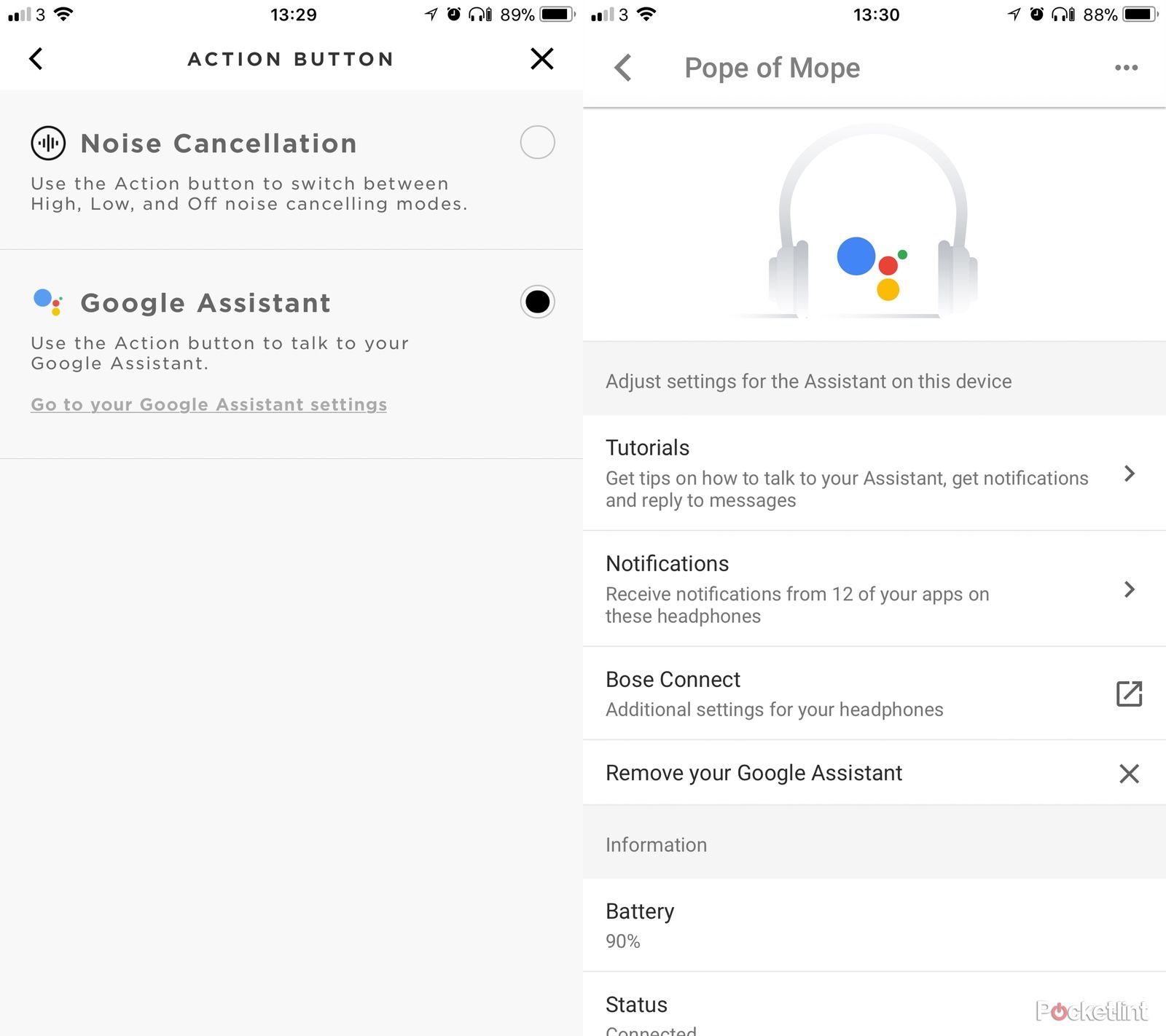**Descriptive Caption:**

"This image depicts a user's smartphone interface with various connectivity and settings details. At two different times, 13:29 and 13:30, the phone displays 2 out of 4 cellular signal bars and full Wi-Fi connectivity. The battery levels indicated are 89% and 99%, respectively, with various device functions such as location services, clock, and headphones being active.

The screen provides information on noise cancellation options, which can be adjusted using the action button to switch between high, low, and off modes. The Google Assistant is prominently featured, offering tutorials, tips, and settings adjustments for ease of use. Notifications for both a 12-ounce and a cell phone device are present, alongside an adjustable recommendation to remove your Google Assistant if needed.

The battery icon confirms a significant charge at 90%, with the status showing as connected, and mentions of 'pocket lint' suggesting some user humor or context. The action button allows for voice interactions with the Google Assistant, while GPS and other settings remain adjustable on the smartphone. The user interface also highlights functionality for pitch changes via the power button, demonstrating intricate control over device settings and voice assistant interactions."